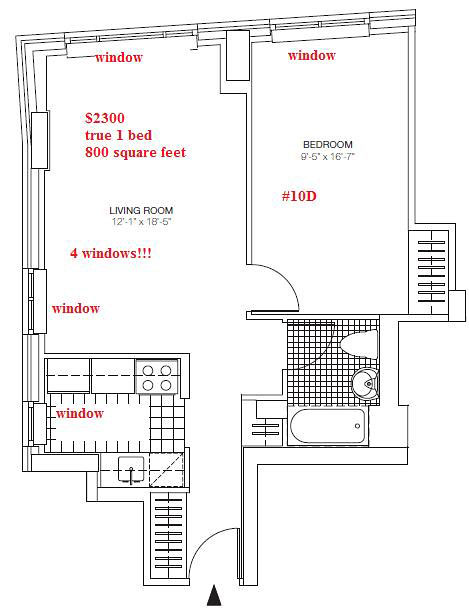This detailed black-and-white floor plan illustrates the entire layout of the apartment, starting from the entryway at the bottom and extending through to the back. At the entrance, there's a small entryway leading directly into the kitchen, which is precisely mapped out. Adjacent to the kitchen is the bathroom. 

Moving further into the apartment, the living room is generously illuminated by four windows, offering abundant natural light. A descriptive label on the image notes that the apartment is a true one-bedroom unit, spanning 800 square feet and priced at $2,300 per month. 

To the right of the living room, the bedroom is shown with detailed dimensions of approximately 9 feet by 6 feet and 16 feet by 7 feet, providing ample space for comfort. The bedroom features direct access to a small patio, ideal for outdoor relaxation. Additionally, a closet is conveniently located within the bedroom, ensuring ample storage space.

Overall, this comprehensive floor plan effectively captures all key elements of the apartment's layout, giving a clear understanding of the space and its features.